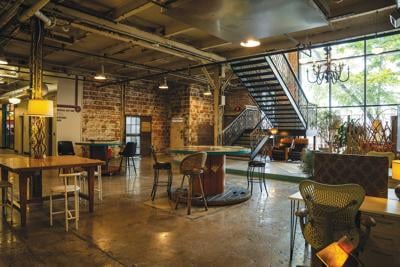This photograph captures the interior of what appears to be a transformed industrial space, possibly a repurposed warehouse, now serving as a modern and eclectic communal area. The room features a large window with lush green trees visible outside, allowing ample natural light to pour in. The floor is a mix of concrete and decorative tile, providing a stylish yet functional base for the various seating areas.

The space is adorned with a collection of furniture that includes round tables made from large spools, commonly used for holding wire or cable, surrounded by unique, ornate bar stools and a mix of regular dining chairs. There is a prominent staircase with wrought iron railings leading to an upstairs area, emphasizing the character of the building. The architectural elements, such as exposed beams, pipes, vents, and soffits, highlight the room's vintage industrial roots.

A notable feature is the large, rustic-looking brick wall that adds to the cozy, yet industrial ambiance. Scattered throughout the room are various lamps, both hanging from the ceiling and placed on tables, providing warm, inviting lighting. Track lighting on the ceiling and a candelabra chandelier further illuminate the space, enhancing its eclectic decor.

In addition to the different seating arrangements, there's an L-shaped bar built around one of the structural pipes, contributing to the room's unique and dynamic layout. Various tables, including square, angular, and bar-like surfaces, offer multiple spots for working, reading, or simply hanging out. The eclectic mix of furniture and decor, combined with the room's vintage-industrial aesthetic, creates a beautiful, comfortable, and collaborative environment.